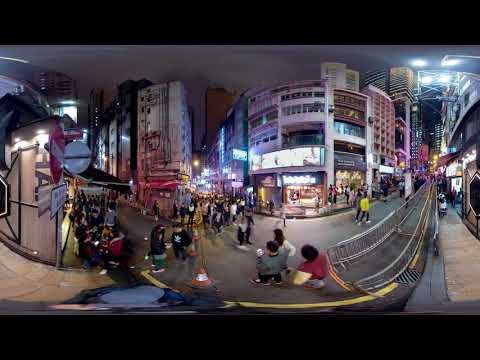This color photograph, presented in landscape orientation with a black border along the top and bottom, is a composite panoramic image combining three different perspectives of a bustling nighttime city scene. The scene appears slightly distorted, creating a stretched arc effect reminiscent of a bent mirror. The central focus is on the street life, teeming with people walking and milling around, with many seemingly waiting in line, possibly to enter a store. Among the background of tall commercial buildings are brightly lit neon signs in hues of pink, yellow, white, and blue, contributing to the lively atmosphere.

On the right side of the image, temporary pedestrian fences line a sidewalk that extends deep into the background, while yellow lines painted on the road suggest the presence of public transportation. The buildings, although closely packed and towering, display varying states of upkeep, with some adorned with graffiti and noticeable cracks. The left segment of the panorama shows a retail shopping area at dusk, dimly lit but still bustling with activity. The central segment offers a different perspective of this same area, focusing on a six-story retail building with other skyscrapers receding into the distance. The right segment highlights a wood sidewalk running alongside the street, providing a more focused view of the pedestrian flow in front of the shops. The photographic style is a blend of representationalism, realism, and panoramic imagery, collectively presenting a vivid and detailed snapshot of urban nightlife.